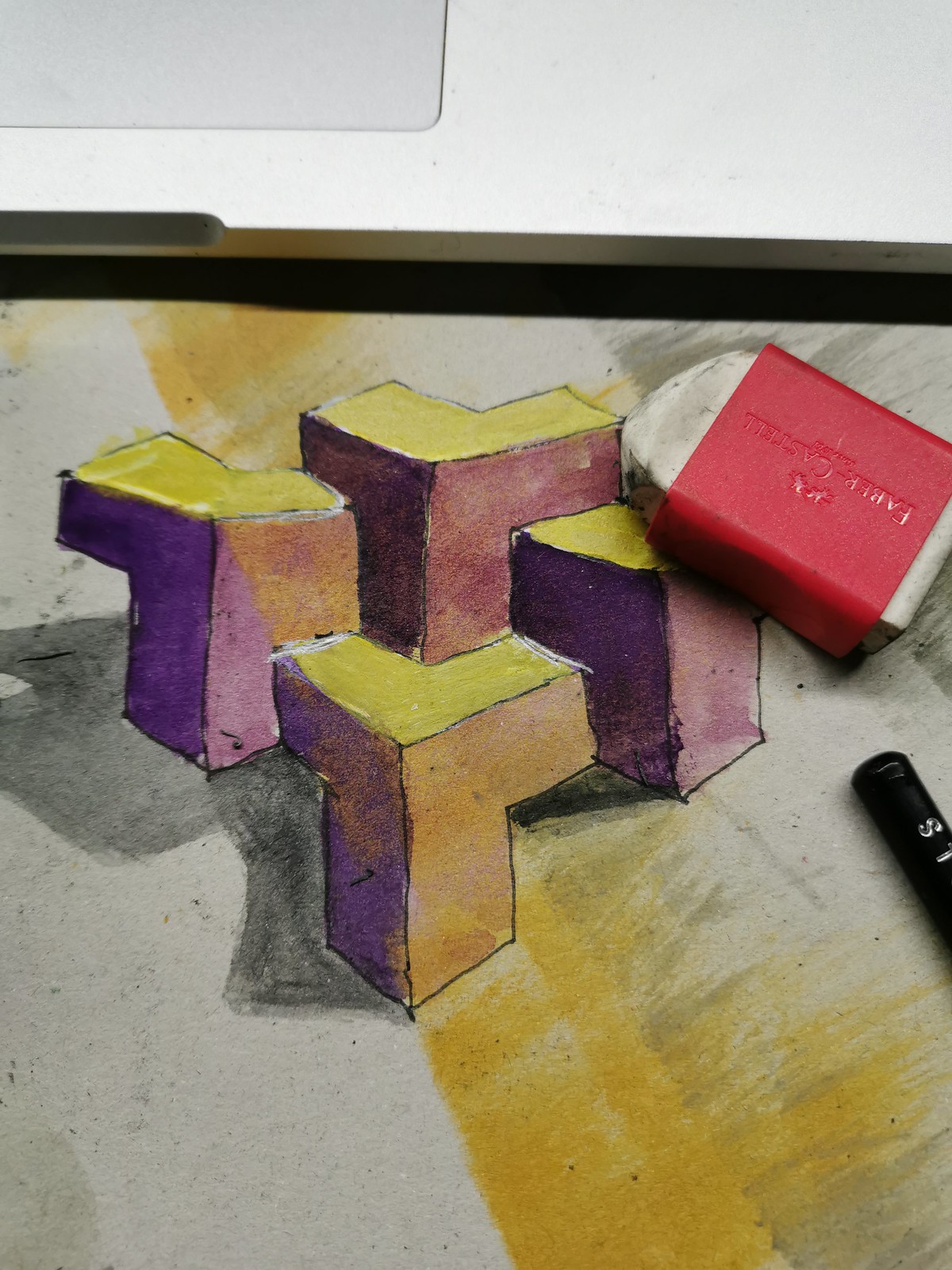This image captures a detailed photograph of a pencil drawing or pastel sketch rendered on a paper surface. Central to the artwork are several three-dimensional Y-shaped or T-shaped linear structures, each meticulously shaded to enhance their 3D appearance. The tops of these shapes are primarily yellow, transitioning into purple, pink, or orange hues down their sides, with gray shading accentuating their depth. The background consists of a blend of darker and lighter gray tones, complemented by streaks of brown and more subtle yellow and gray shadings near the bottom. 

In addition to the drawing, an eraser with a red plastic sleeve is positioned near the top portion of the artwork. This white eraser shows signs of use, with rounded-off edges. Adjacent to the eraser is the tip of a black pencil or marker, possibly marked with the number 8 or the letter S in white. The composition is framed by the elegant interplay of colors and shadows, creating a visually compelling portrayal of the artist's tools and creative process.